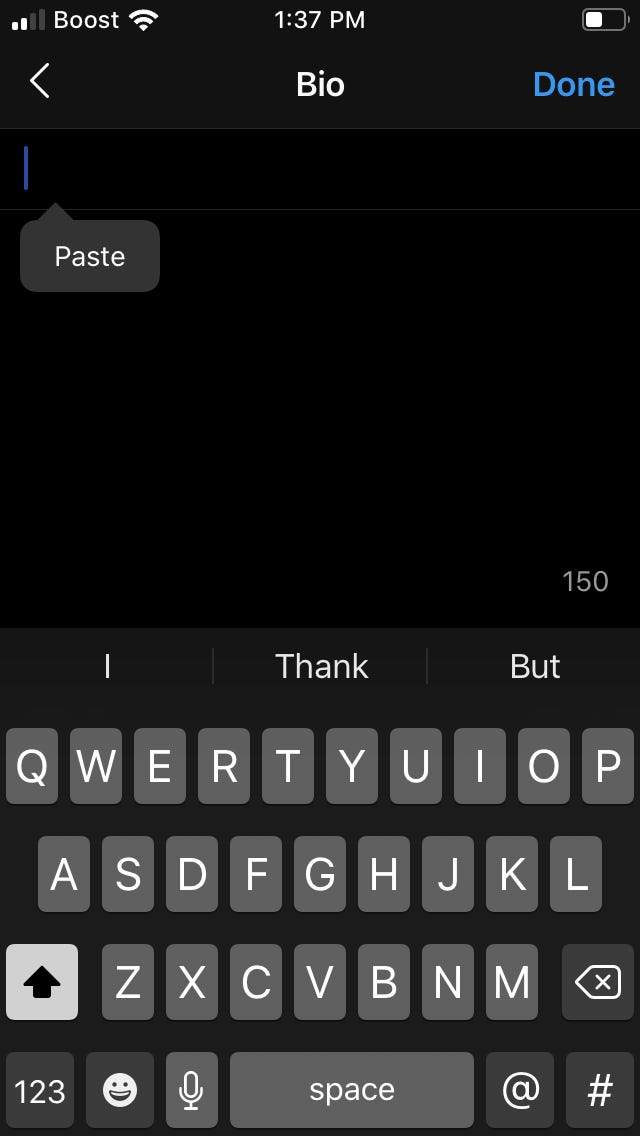The image displays the screen of a device with a black background and predominantly white text. Notably, the word "Done," written in blue, is located at the top right corner. On the top left, a series of icons are visible, starting with a cellular signal icon followed by "Boost," then a Wi-Fi signal icon. Centrally positioned at the top, the time reads 1:37 p.m. To the top right, a battery icon shows that it is approximately half full.

Just below the top bar on the left side, there's a left-pointing arrow. Centrally, the word "Bio" is displayed, and to the right is again the word "Done." Further below on the left, the word "Pace," spelled P-A-S-T, is visible. This is followed by three sections: the leftmost section reads "I," the middle section says "Thanks," and the rightmost section reads "But." Below these sections, an image of a keyboard with letters is prominently displayed.